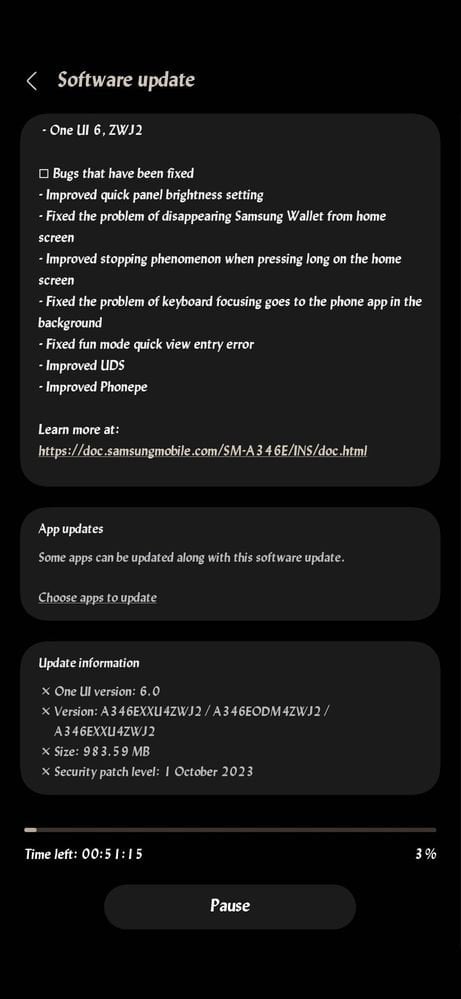**Software Update Page on a Samsung Device**

The image showcases a black web page detailing the software update information. The entire background is black with white text prominently displayed at the top, reading "Software Update." Below this heading, the current software version is listed as "1Lii6.zwj2."

Underneath, there is a bulleted list of updates and improvements:
- Bug fixes
- Improved Quick Panel brightness setting
- Resolved issue with Samsung Wallet disappearing from the home screen
- Enhanced response to long presses on the home screen
- Fixed problem where the keyboard focus switches to the phone app in the background
- Corrected "Fun Mode" Quick View entry error
- Improved UDS functionality
- Enhanced Phone PE performance

A link to more detailed information is provided: "Learn more at https://doc.samsungmobile.com/sm-a3460-ins/doc.html."

The page then moves to an "App Updates" section, stating that some apps can be updated along with the software. Users are prompted to choose which apps to update.

Further down, another section presents "Update Information":
- Software Version: 1Lii, 6.0, a360xxu4zwj2/a3460odm4zwj2/a3460xxu4zwj2
- Size: 983.59 MB
- Security Patch Level: 1 October 2023

At the bottom, there is a progress bar indicating the update status. The bar shows time remaining as "00:51:15," indicating 3% completed. Below the progress bar, there is a pause button.